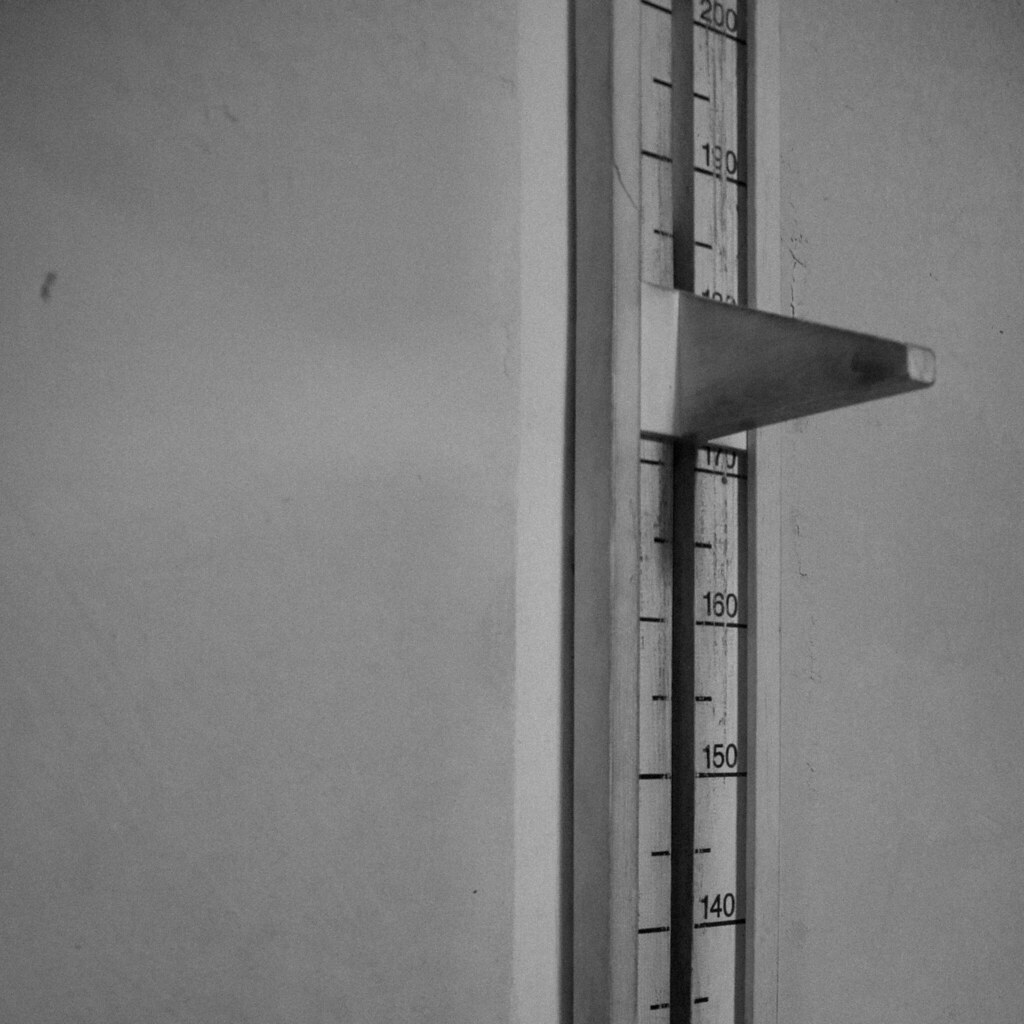This black-and-white photograph captures a height measurement gauge mounted on a light-colored wall. The gauge is vertically aligned with markings in intervals of 10, ranging from 140 at the bottom to 200 at the top, suggesting it measures height in centimeters. The numbers are distinctly printed in black, possibly on a white background, providing a stark contrast that enhances legibility. A metallic component protrudes horizontally from the gauge, indicating it could be designed to rest on top of a person's head to measure their height accurately. The overall composition is stark and minimalistic, emphasizing the functional yet industrial design of the measuring instrument. The photograph's monochromatic nature highlights the textures and contrasts within the scene, drawing attention to the gauge's precise detailing and utilitarian purpose.